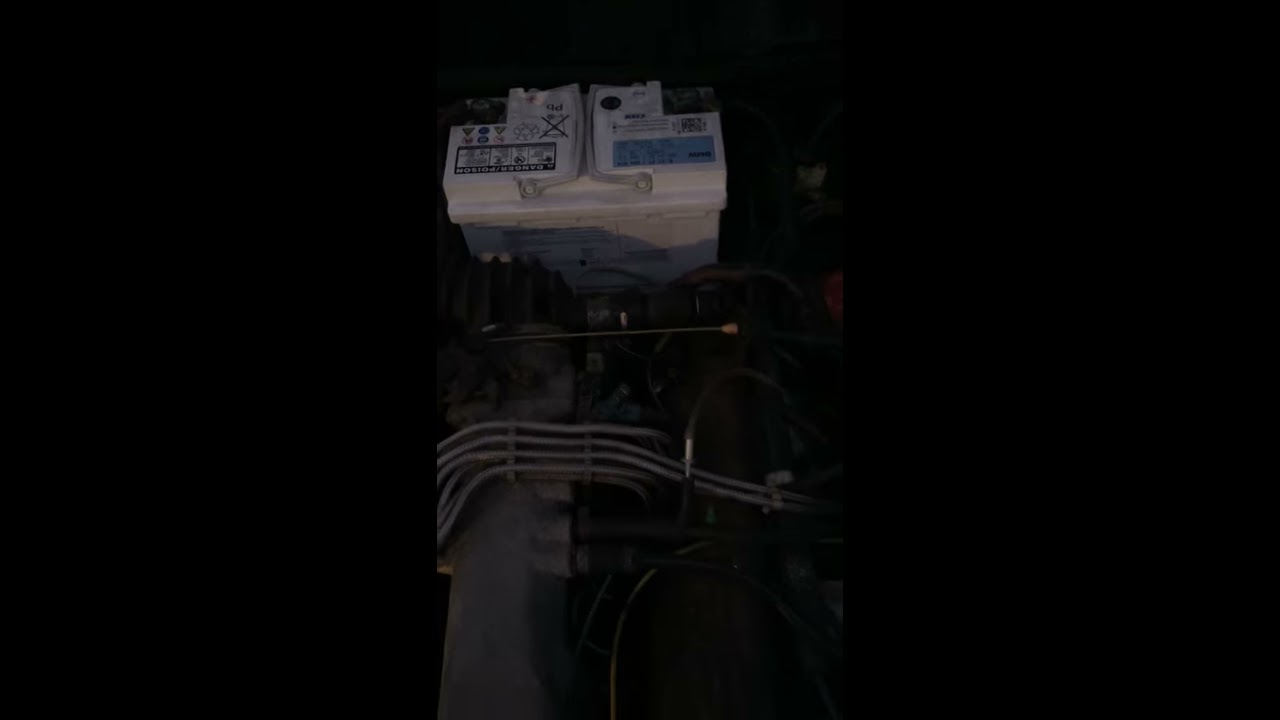The image is a horizontal rectangular photo predominantly showcasing a dark setting, possibly outdoors at night. Central to the image are two cylindrical metal components: the one on the left is light gray while the one on the right is a very dark gray. These metal cylinders are interconnected by a network of black and gray cords. Positioned above these cylinders is a prominent white rectangular canister with what appear to be hazard labels featuring the letters "GD" alongside a large crossed-out symbol. This canister, resembling a car battery but distinctively white, features small black knobs and various writings and diagrams upon its surface. Surrounding the main components, additional wirings and engine-like elements suggest that the scene is a close-up view of an engine bay, viewed from above.